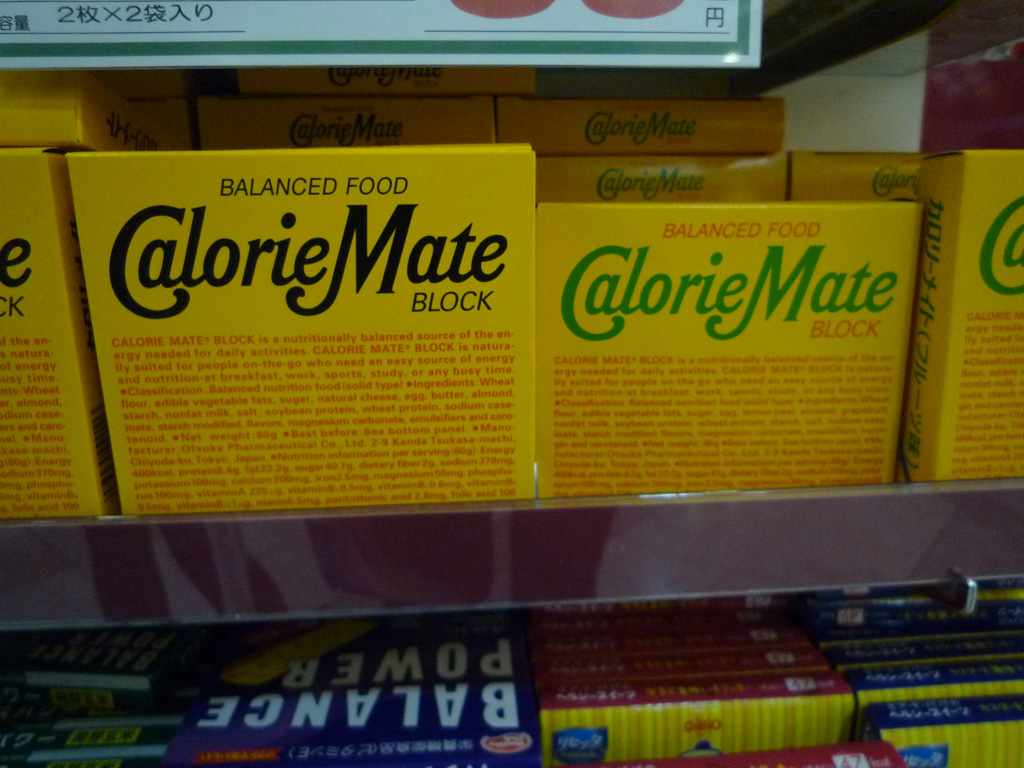A well-organized shelf in a store presents an array of uniformly lined-up items. The shelving unit, primarily made of metal, is partially visible, running horizontally and sectioned off in the image's lower center. The shelf displays only a segment of the items on the next tier below. Meanwhile, at the top of the image, the shelf extends almost entirely from the left to right. A price tag sign is discernable towards the left. The focal point of the image is prominently small boxes of a product named "Calorie Mate," with one box showing its back facing outward.